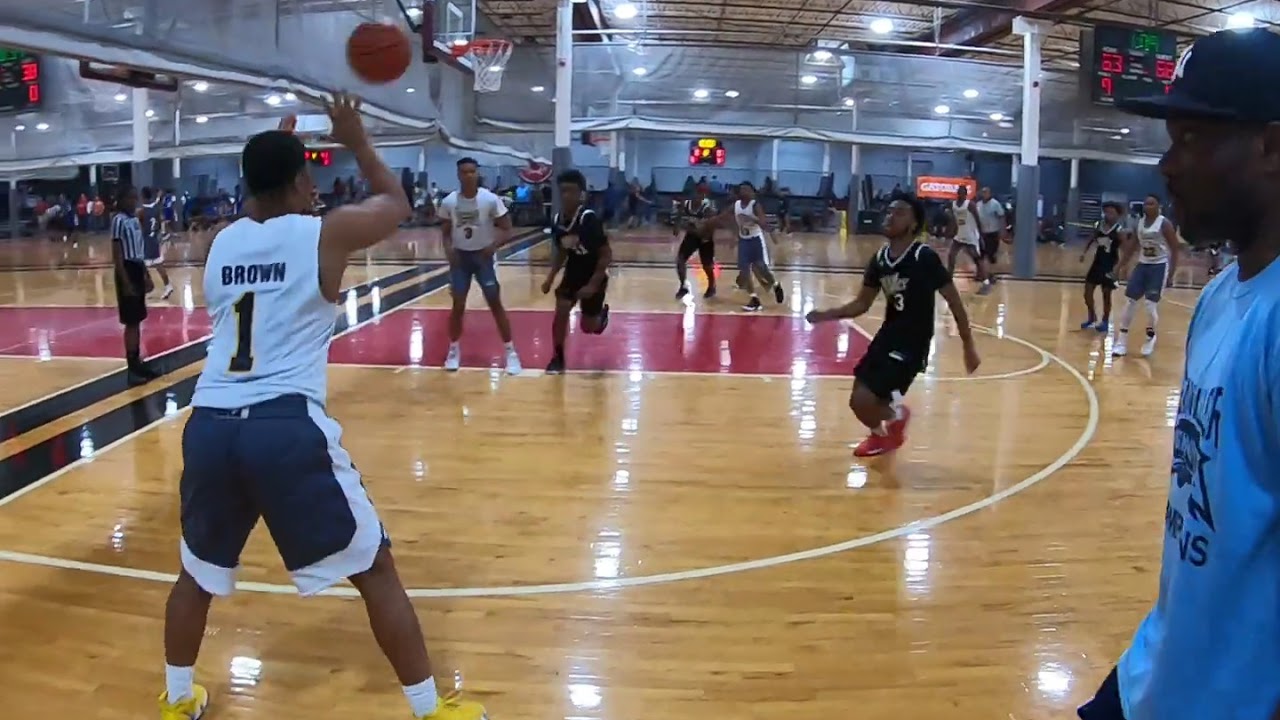The image captures a lively scene inside a large gymnasium, where multiple organized basketball games are taking place simultaneously. The gym features a hardwood floor, with a distinct red-painted area directly underneath the basketball hoops. White arcs and three-point lines are clearly visible on the court.

In the foreground, a young player in a white jersey, identified by "BROWN" and the number one on his back, stands near the three-point line, either receiving or preparing to shoot the basketball. He is dressed in blue shorts with white trims, white socks, and yellow shoes. On the left side of the frame, a man in a blue shirt and black cap is staring at Brown, while two players in black jerseys and shorts approach him. 

Another player with a white jersey and the number three stands beneath the hoop in the background. The gym's upper right corner features a scoreboard displaying a score of 63 to 62, and another scoreboard can be seen further back in the middle of the picture. The gym's ceiling is adorned with light-translucent tarp barriers, allowing the illumination to shine through.

Interestingly, the gym walls are mirrored, adding a unique visual element to the scene. A referee is visible on the court, underscoring the organized nature of the games.